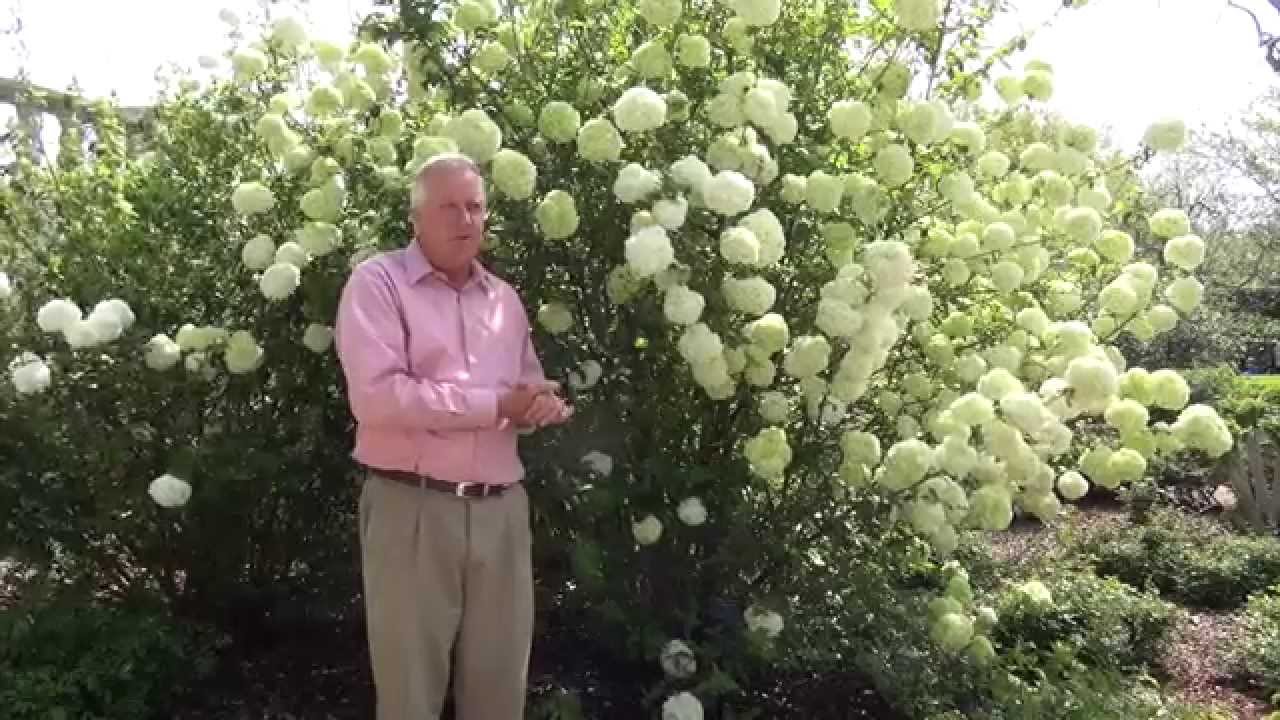The photograph features an older white man, likely in his late 50s to 60s, with receding gray hair and a facial expression of curiosity. He is dressed in a long-sleeved pink business casual shirt, khaki pleated pants, and a brown leather belt. His hands are clasped together. The man stands in front of a towering bush, approximately 8 to 10 feet tall, covered in numerous white flowers that resemble pom-poms or snowballs, possibly roses or mums. The bush has vibrant green foliage, and various other shrubs and trees are visible in the background. The ground around him is woody and root-filled, contributing to the lush, botanical setting. The sky overhead is unusually bright, appearing as a washed-out yellowish white, adding an ethereal quality to the scene. The man, likely a proud gardener or an enthusiastic visitor to a botanical garden, stands centrally in the image, with the tall, flower-laden bush creating a striking backdrop.